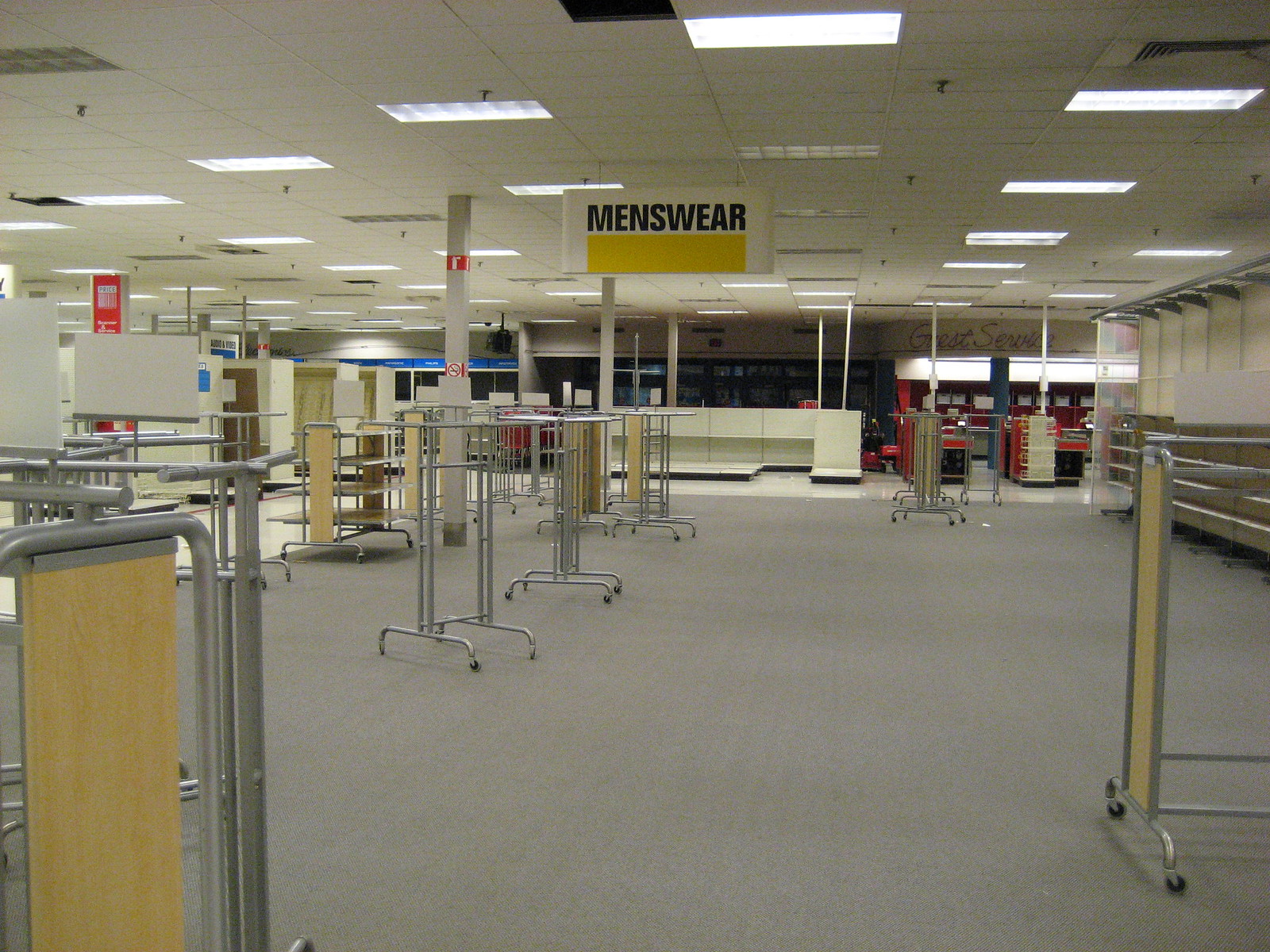The photograph depicts an abandoned or emptied department store section, most likely due to the store either going out of business or in the process of closing down. The floor is covered in a gray carpet, and scattered throughout the space are empty metal racks, many on small roller wheels, along with shelves featuring light wooden sides. Dominating the center top of the image is a rectangular sign suspended from the white ceiling, which houses common rectangular-shaped lights; the sign, reading "MENSWEAR" in bold black capital letters atop a yellow rectangle, signifies that this area was once designated for men's clothing. In the backdrop of the image lies an all-glass entrance, while the environment is dotted with white poles and red-and-white "NO SMOKING" signs. The arrangement of the depleted racks and barren shelves underscores the store's desolation. The color palette primarily features shades of black, white, and yellow, with glimpses of red adding minor accents throughout the scene.